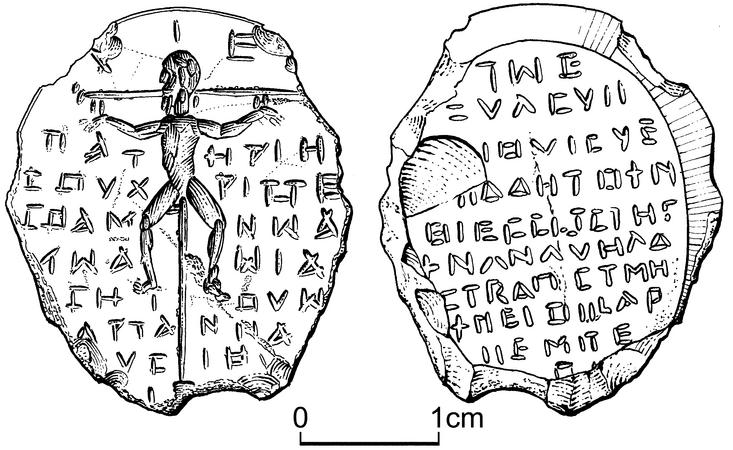This black and white image features two roughly circular, uneven and jagged edged stones that are each only a few centimeters in diameter, as indicated by the 0-1 cm measuring scale at the bottom of the image. The background is white. The stone on the left bears what appears to be a rudimentary human figure positioned as though balancing on two fingers of each hand, evoking the appearance of a figure on a cross. This stone also features carved text resembling characters, some identified as NWPIH, though they are not the typical English alphabet and lack any curved shapes, with the 'P' resembling a triangle. The stone on the right shows similar irregular text with a prominent central dome shape, surrounded by a rough circular border within the larger stone's shape. Both stones appear to be artifacts with carvings that might be Cretan in origin, reflecting ancient or rudimentary script.